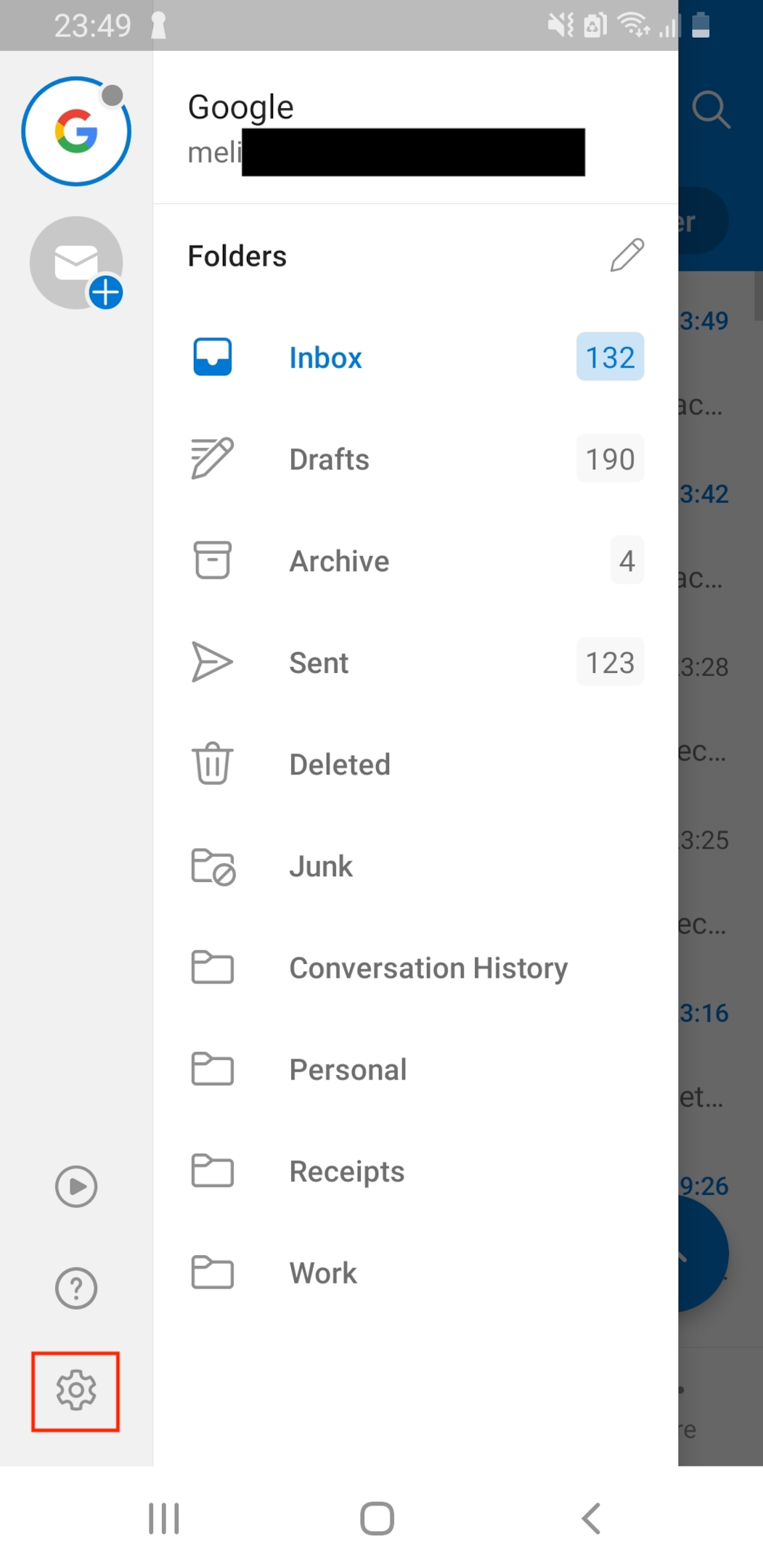Screenshot of a Google email account interface displaying the time "23:49." The sender is identified as "Google," with the email address partially redacted to "MBL...". The left sidebar features a list of folders, each accompanied by a distinct icon. These folders include:

- **Inbox** (132 emails)
- **Drafts** (190 emails)
- **Archive** (4 emails)
- **Sent** (123 emails)
- **Deleted**
- **Junk**
- **Conversation History**
- **Personal**
- **Receipts**
- **Work**

A red box highlights the settings icon, situated below a circled question mark icon and a circled play button icon. The interface background is primarily white and gray, accented with some blue text.